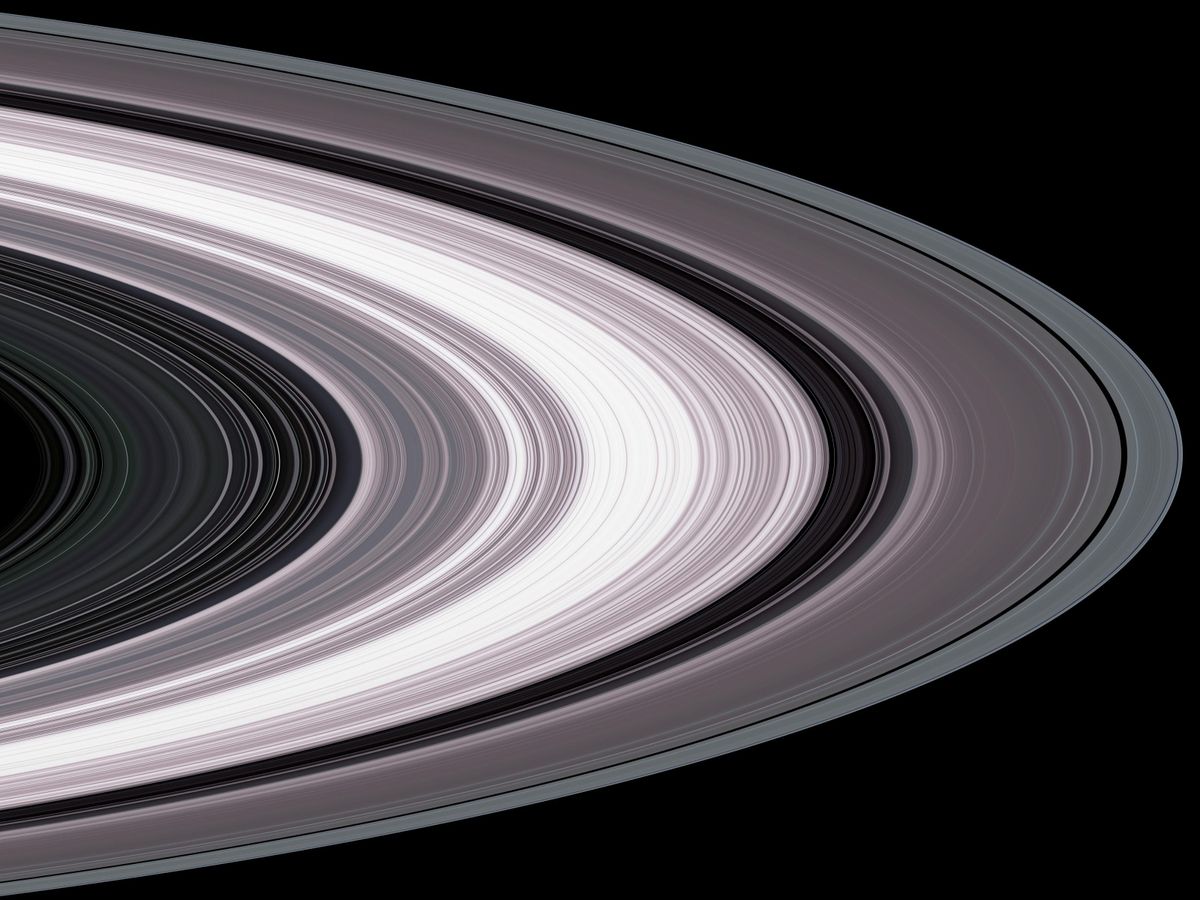The image depicts the intricate rings of a planet, reminiscent of Saturn, set against a stark black background. The rings display a diverse palette of colors and bands. The outermost layer is a dark gray, transitioning inward to a dark brown layer with bands of lighter colors, including pink, red, and even green. Further in, a very sparse segment precedes a pronounced thick white layer, followed by another sparse area. Numerous distinct layers are visible, combining shades of brown, black, gray, purple, and even a very dark violet, arranged in a pattern of arcs. Despite the high saturation of colors, the depiction remains somewhat stylized and digital, suggesting a creative interpretation rather than a realistic photograph. The entire arrangement, from thick to sparse bands, contributes to a visually captivating portrayal of planetary rings in outer space.